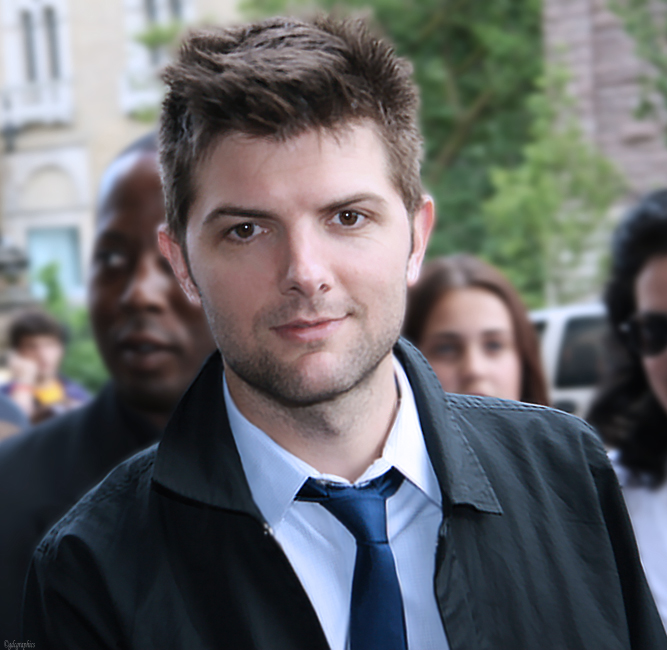In this photograph, actor Adam Scott is pictured, likely taken a few years ago during a daytime event or publicity appearance for a movie. Adam features short, spiked brown hair, brown eyes, and a slightly unshaven look with a bit more than a five o'clock shadow. He is dressed in a gray long-sleeve jacket made of a raincoat-like material, paired with a white collared dress shirt and a turquoise or blue-green metallic sheen tie.

Behind Adam, the background is slightly blurred, but it includes several individuals and elements. To his left (the right side of the photo), there are two women with brown hair, one of them having slightly reddish-brown hair and hair down to her chin. To his right (the left side of the photo), there is a black man looking to his right, out of the frame. Additionally, a person with dark black hair and wearing sunglasses is partly cut off on the far right side.

In the distance, a man can be seen on a cell phone, and there is a white SUV or truck visible with a large window and door handle. The scene is set against a backdrop of brick and stone buildings interspersed with green trees, indicating a setting perhaps in a city or a suburban area.